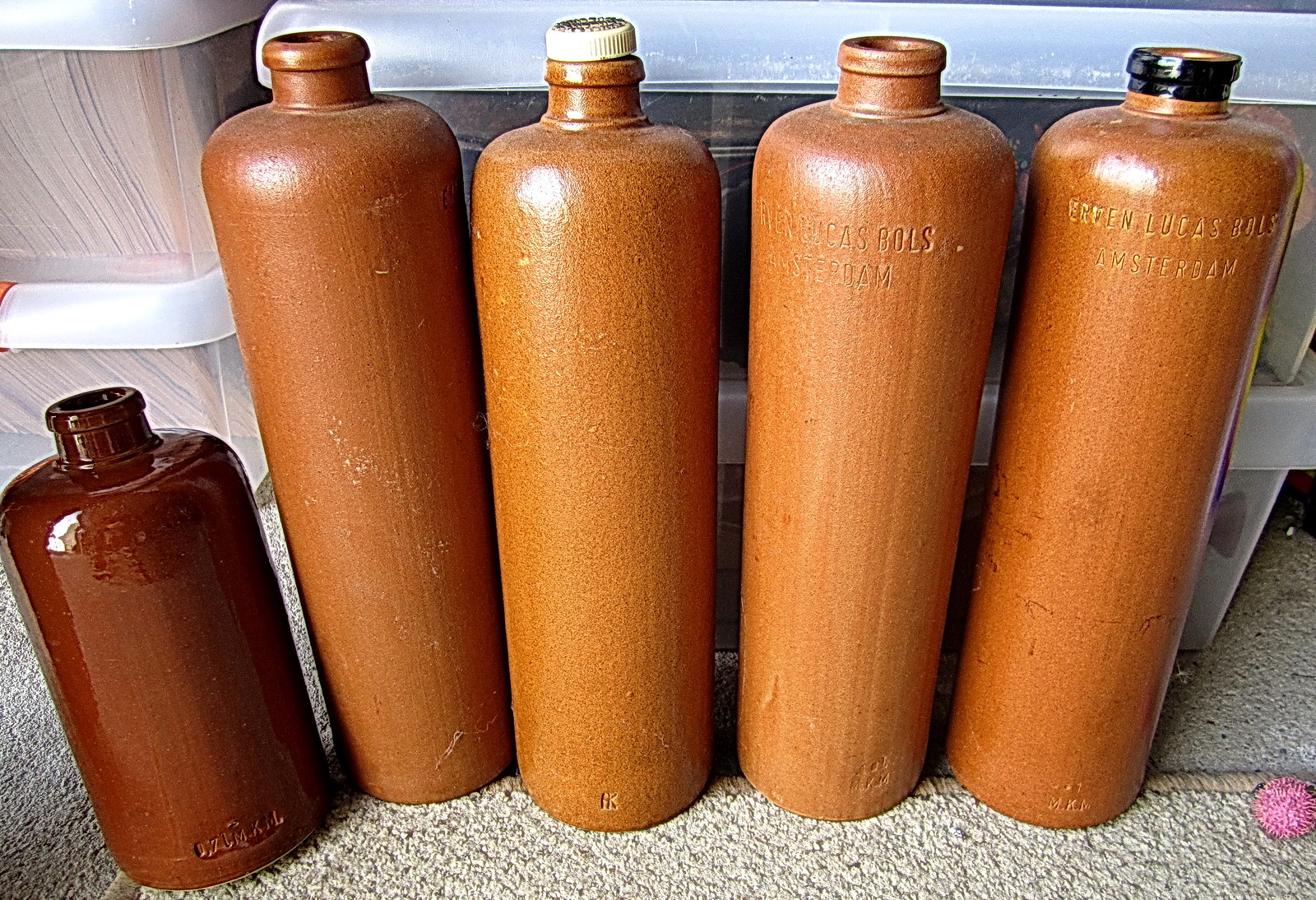The indoor photograph features a collection of pottery bottles, meticulously arranged on a beige and white carpet. In the forefront, there are four tall, terracotta pottery bottles, each resembling the size of wine bottles but with distinctive squared, rounded shoulders. The bottles prominently exhibit engraved text; the rightmost bottle is particularly notable, displaying the inscription "Ervin Lucas B-O-L-S" followed by "Amsterdam." Among these, the second bottle also features a contrasting white cap, while the others remain open at the top. On the far left, a noticeably shorter and slightly wider bottle stands out with its darker, glossy brown finish. Surrounding the pottery bottles is a scattered arrangement of items: a plush, pink cat toy ball on the bottom right and several clear plastic storage boxes to the upper left containing manila file folders.